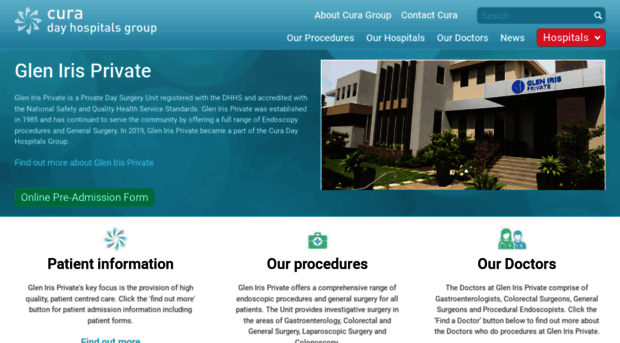The screenshot displays a section of the Cura Day Hospitals Group website. At the top is a wide banner with a gradient background transitioning from light blue to dark blue. The banner features the Cura logo, which consists of swirling drops forming a circle. Text within the banner reads "Cura Day Hospitals Group." To the right are links labeled "About Cura Group" and "Contact Cura," followed by a search bar.

Below the banner, a navigation menu includes the options: "Our Procedures," "Our Hospitals," "Our Doctors," and "News." A distinctive red button labeled "Hospitals" indicates a drop-down menu for more options.

On the left side of the screenshot, there is a reference to "Glen Iris Private," one of the hospitals within the group. To the right, an image shows the entrance of Glen Iris Private with its name displayed prominently. Accompanying the image is a descriptive paragraph about Glen Iris Private. Below this paragraph, a green button labeled "Online Pre-Admission Form" invites users to start the admission process. 

Additionally, three options are listed at the bottom for further information: "Information," "Our Procedures," and "Our Doctors." This screenshot represents a healthcare website providing detailed information about the Cura Day Hospitals Group and their services.